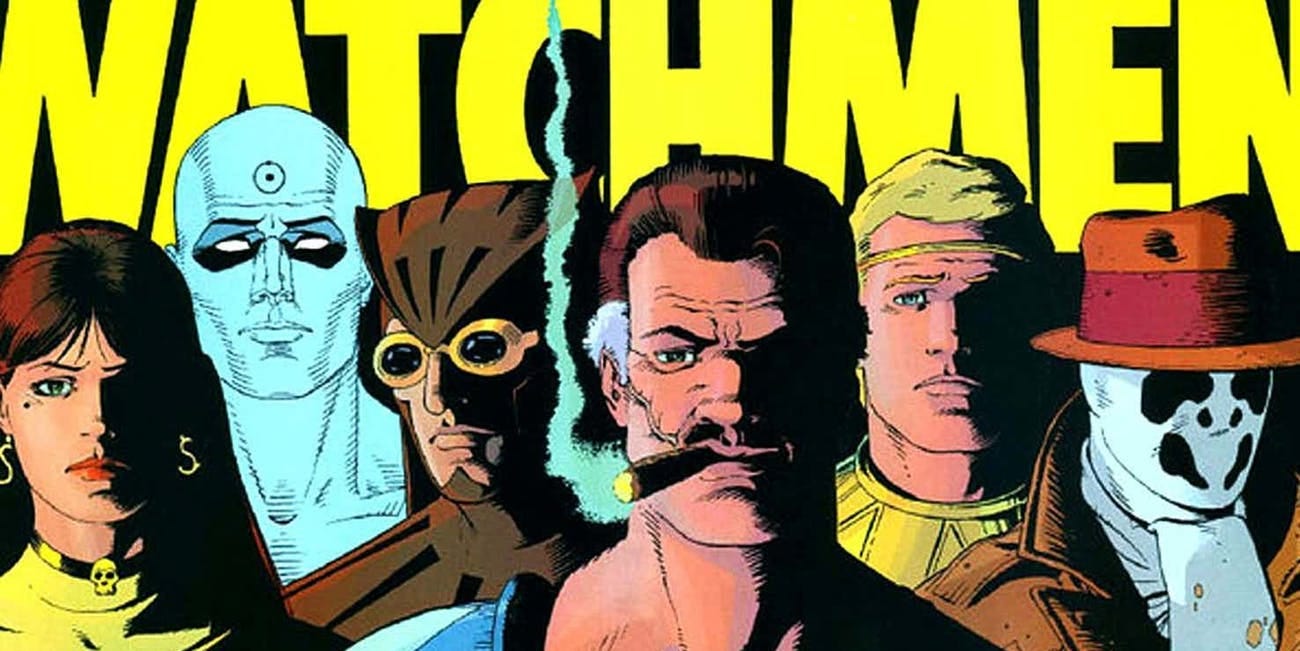This landscape-oriented comic book illustration features six distinct characters lined up from the chest up, set against a black background. The top of the image showcases bold yellow capital letters reading "WATCHMEN," slightly trimmed at the top edge. Starting from the left, the first character is a woman with long dark brown hair, light skin, and a yellow tight outfit. She sports a yellow skull necklace and S-shaped earrings. Beside her stands a ghostly all-blue man with white, blank eyes and a bullseye symbol on his forehead. Next is a man dressed in an owl-themed costume, with gold goggles and a hooded hat, staring to the left. In the center, a tough-looking man in his late forties is seen puffing on a cigar, characterized by his distinctive star-shaped scar. To his right, a younger, blonde man with a gold headband, resembling a Greek god, gazes upward to the left. The final character on the far right is a man wearing a brown fedora, a brown trench coat, and a white Rorschach mask, giving him a skeletal appearance. The detailed and vibrant comic book art style effectively captures the essence and intrigue of the "WATCHMEN" series.